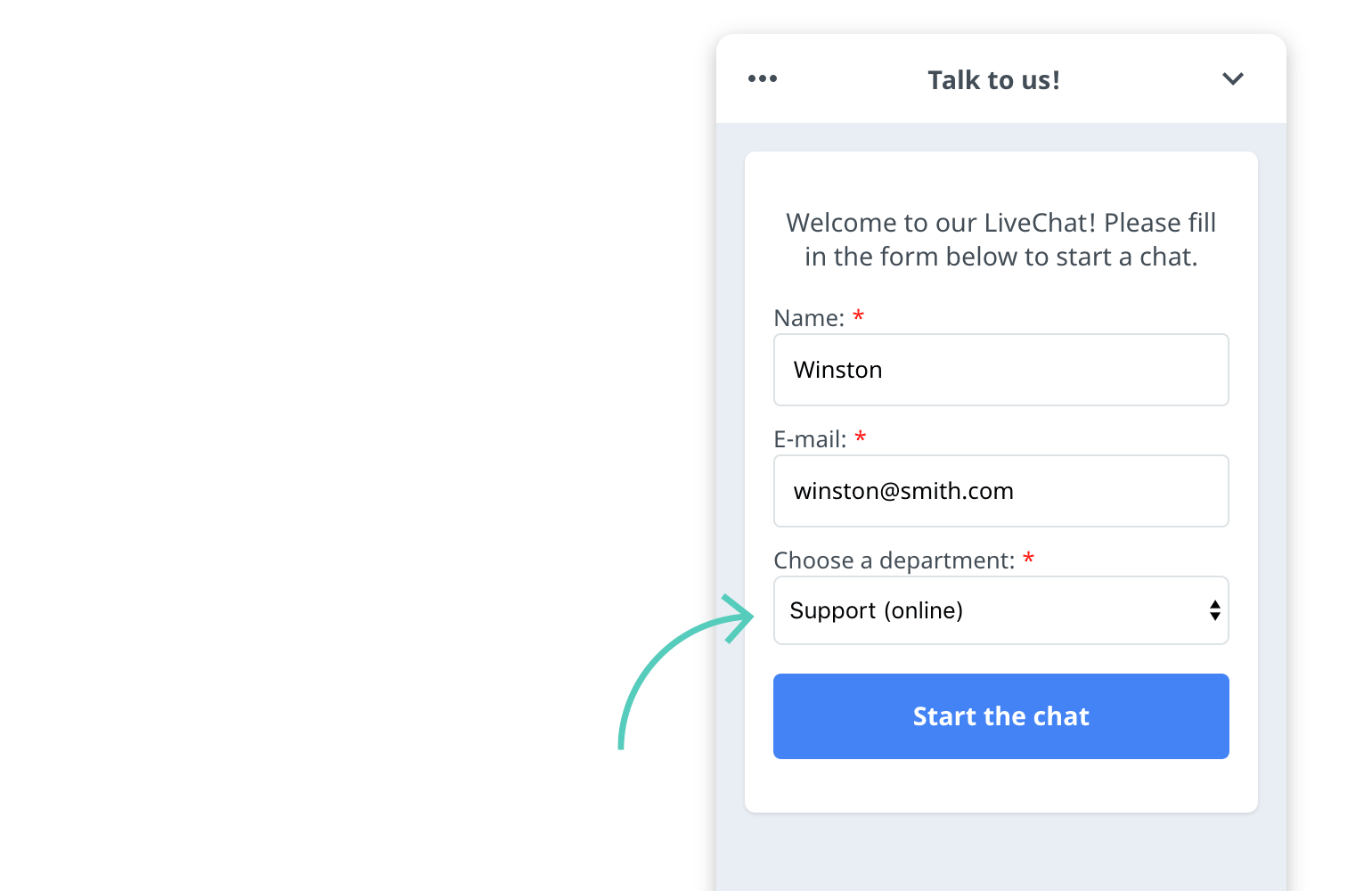In the image, the background is a light blue color, providing a serene and inviting atmosphere. At the top center, there is a white box which contains three small black dots arranged horizontally next to an up and down arrow icon, indicating a collapsible or expandable feature.

Below this, a larger white box dominates the center of the image. This box contains a welcoming message, "Welcome to our live chat. Please fill in the form below to start a chat." Underneath the message, there are fields to collect user information:
1. **Name** - Marked with a small pink asterisk indicating it's a required field, the example text provided inside the box is "Winston."
2. **Email** - Also marked with a pink asterisk, the filled-in example email address is "Winston@smith.com."

Further down, there is a dropdown menu labeled "Choose a department," similarly marked with a pink asterisk. Accompanying this field is a prominent blue arrow pointing towards the option "Support Online," indicating it as the selected department.

Near the bottom of the white box, there is a large, inviting blue button labeled "Start Chat," which users can click to initiate the live chat session.

This live chat interface, featuring Winston's example data, is displayed against the cohesive light blue background. The white and blue color scheme ensures clarity and ease of navigation, enhancing the user experience for those seeking support.